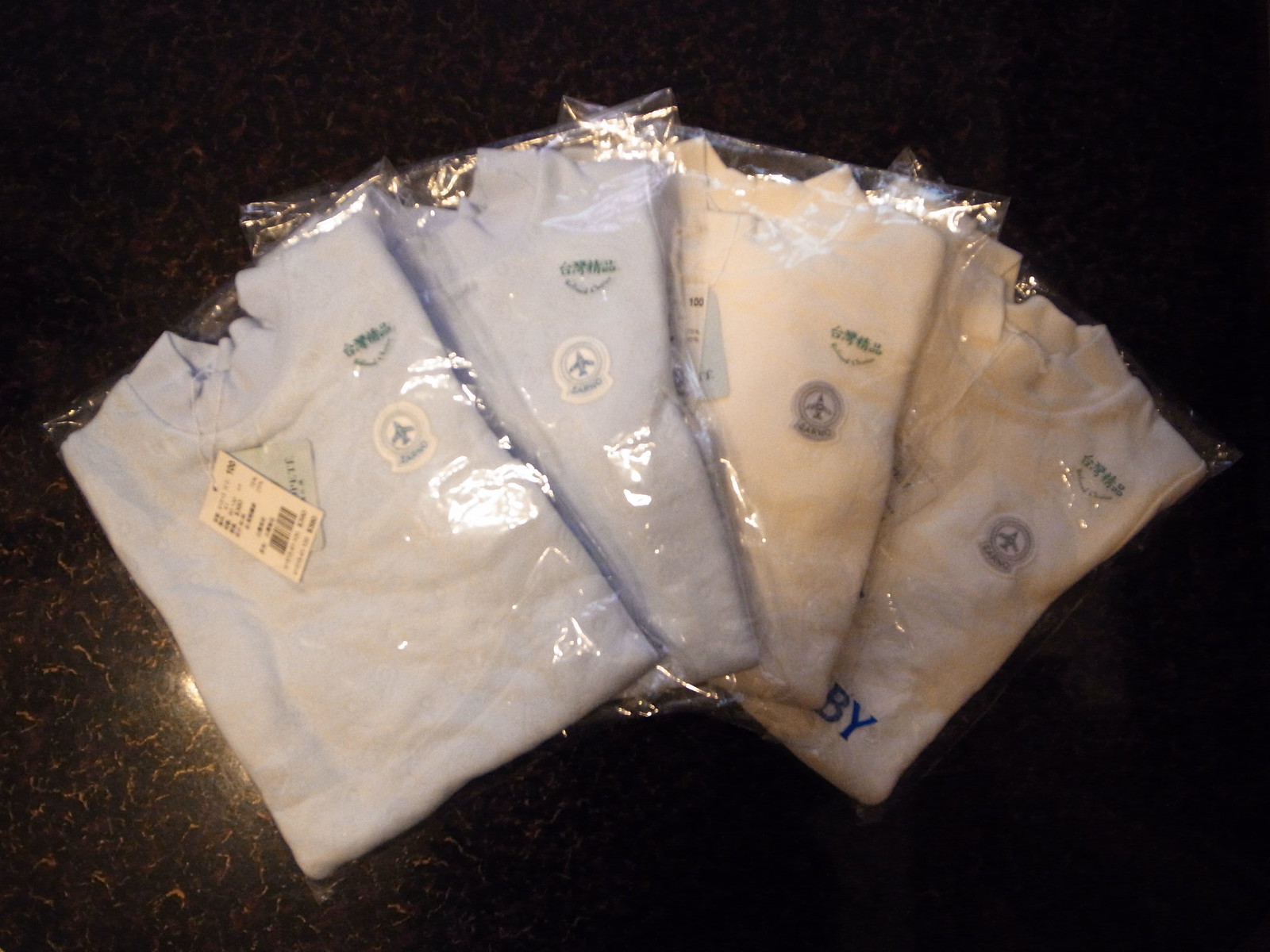This detailed close-up photograph captures four neatly folded and individually wrapped shirts, arranged in a fanned-out pattern on a dark countertop. The shirts are layered from left to right, with the two on the left being light blue and the two on the right being white. Each shirt features a visible store tag, although the details on the tags are not legible. The shirts appear to be long-sleeve and possibly for company use, as they each display identical logos. The black background accentuates the colors of the shirts, suggesting a presentation suitable for online retail or display.